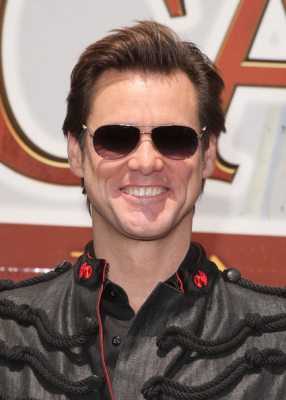This vibrant color close-up photo captures a young Jim Carrey with short, neatly combed brown hair and no gray, revealing his forehead. He's sporting dark brown aviator sunglasses, flashing a big, toothy smile. Carrey's attire is a striking gray jacket, detailed with black cords running across the front, complemented by a black trim around the top and red buttons on each side, along with a noticeable red zipper. Behind him, partially obscured, stands a sign featuring the large letters "C" and "A" in a red hue against white, with the surrounding wall tinged in an orangey-brown color. The overall cheerful demeanor and 80s vibe are unmistakable, highlighting Carrey's early charm and style.